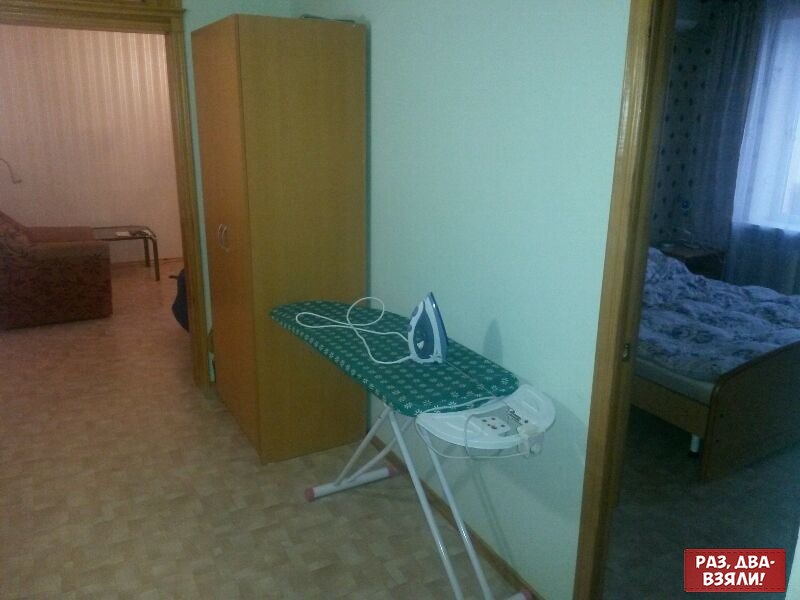This detailed photograph captures the interior of a house that exudes a vintage charm, evocative of the 1970s or 80s. The primary focus is an ironing board set against a light green wall, covered in a turquoise or blue floral pattern, and standing on white legs connected by bars. An iron, with a white and blue design and a white cord, sits upright on the board facing the wall. Surrounding the board, details of two different rooms are visible. To the left, an open sliding door reveals a room with parquet wood flooring and a brown lounge chair with vertical blinds hanging on a window. This room is edged by light wood trim and features a tall, light brown cabinet with brown handles. To the right, another open door frame, also trimmed in brown, leads into a bedroom characterized by a dark, perhaps 70s shag carpeting. A bed is visible along with a window draped in blue chiffon or white sheer curtains, partially open to let in light. The overall decor, including the wallpaper and wooden trim, emphasizes a consistent vintage aesthetic throughout the depicted space.